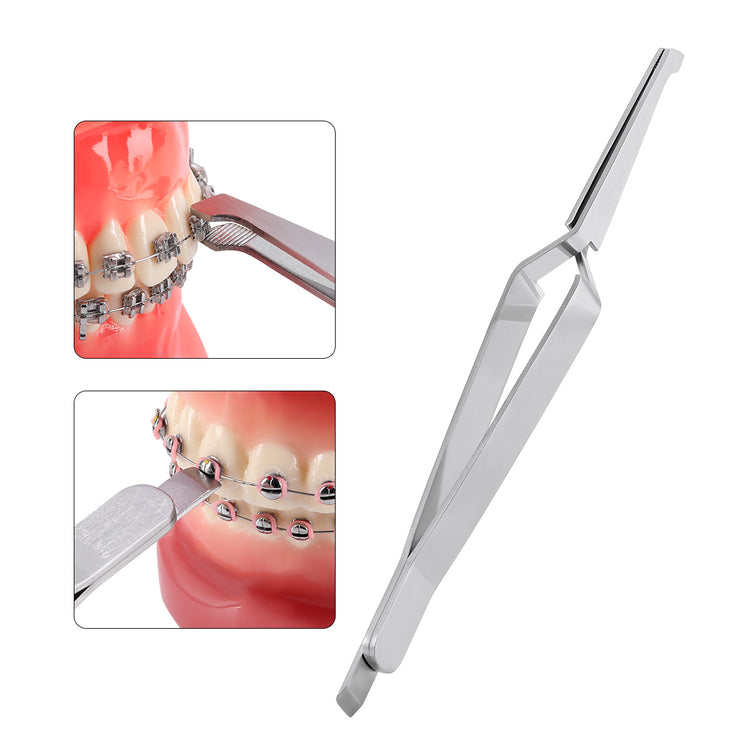The image depicts an orthodontist tool specifically designed for adjusting the brackets on braces. The tool itself is featured prominently on the right side of the image; it resembles elongated tweezers, composed of silver bands with dual functional ends. One end of the tool is equipped with a flat screw tip for making precise adjustments to the brackets, while the opposite end functions as a pinch or wedge tool for similar alterations. On the left side of the image, there are two smaller photos illustrating a simulated mouth with braces. The upper photo shows the bracket adjustment process using the pincher end of the tool, highlighting how the tool interacts with the metal brackets and wires. The lower photo provides a different angle of the procedure, focusing on the screwdriver end positioned under a bracket. These detailed diagrams showcase the practical applications of the tool in a clinical setting, emphasizing how it aids orthodontists in managing and fine-tuning the braces effectively.